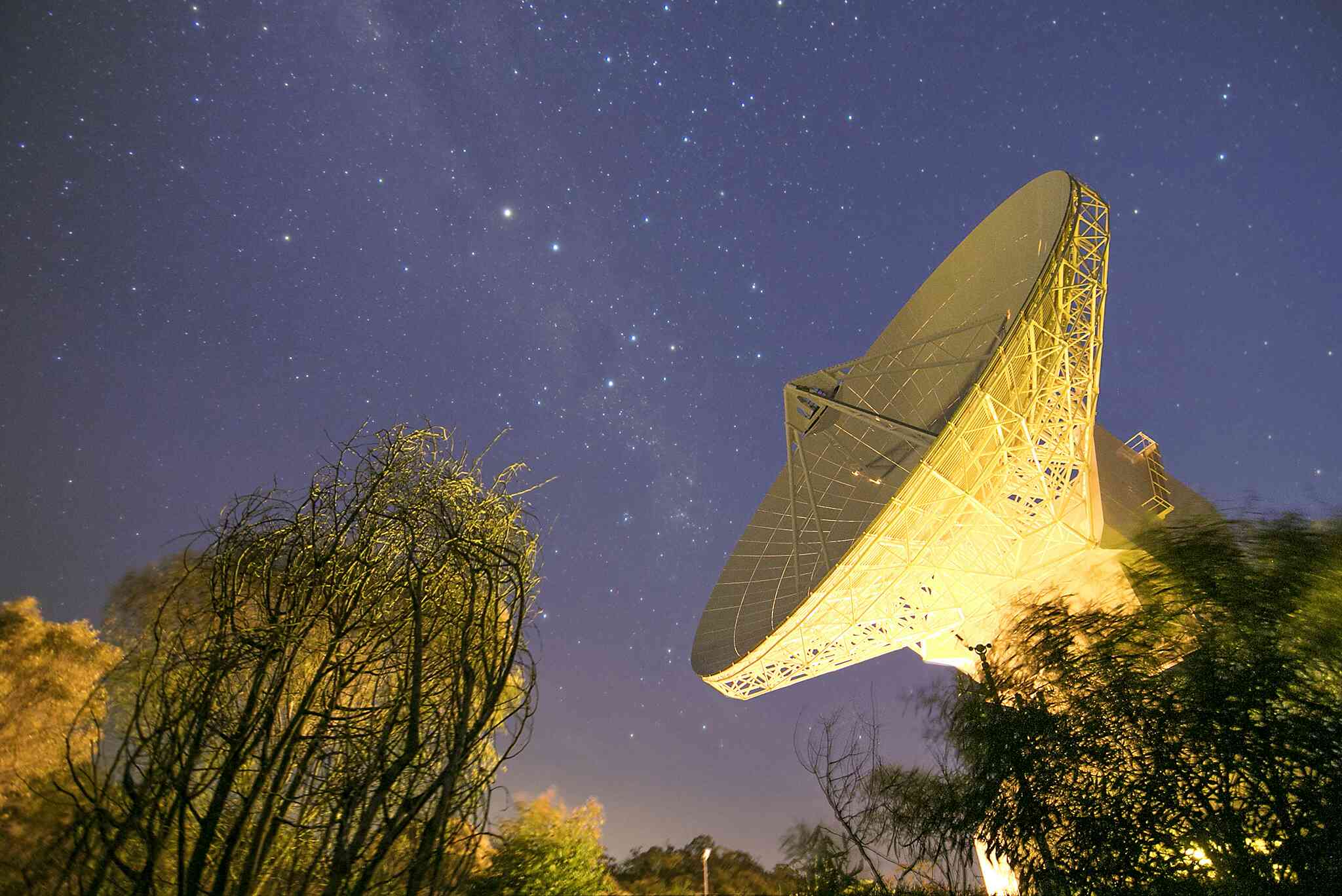In this horizontally aligned rectangular night image, the sky serves as a stunningly speckled backdrop, featuring a pretty gray hue with a tint of purple, adorned with twinkling white stars. Dominating the right side of the picture is a large satellite dish, located in Australia, characterized by its circular shape and pyramid-like center structure. Its surface appears mostly brown and yellow, illuminated by ground lights. The intricate network of metal bars attached to its back is visible as it faces towards the upper left.

In the lower left corner of the image, there is a noticeable cluster of trees, their leaves showcasing a mix of brown and green hues. The vertical branches intriguingly resemble grass attached to them. Similarly, in the lower right corner, another group of trees appears, with their tops slightly blurred, adding to the scene's mystique. The confluence of these elements creates an arresting visual narrative against the star-speckled night sky.